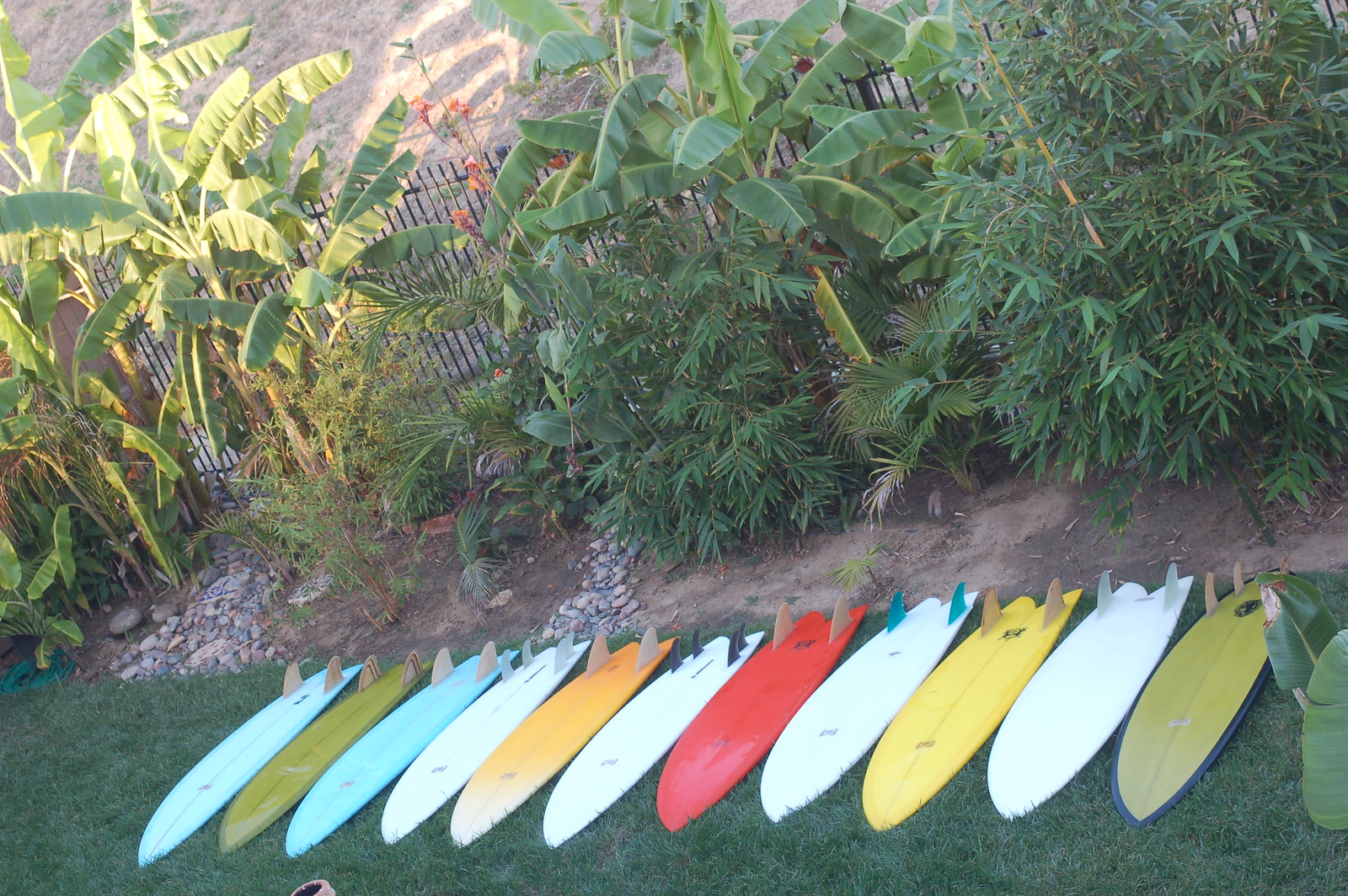In this outdoor photograph, taken from an elevated vantage point possibly a second story, we see 11 surfboards arranged in a neat line lying face down on vibrant green grass, with their twin fins up and the pointed ends angled towards the viewer, roughly oriented around the 6:30 to 7:00 direction. The surfboards feature a spectrum of colors including light blue, dark green, white, orange, red, yellow, and another dark green. Positioned in the bottom third of the image, the array of surfboards is framed by a diverse array of vegetation comprising tropical foliage, bamboos, palm trees, and some shrubbery near a patch of dirt. A modest black metal fence, standing a few feet tall, separates this verdant scene from a brown sandy area beyond it, suggesting proximity to a beach or body of water, under a bright daytime sky.